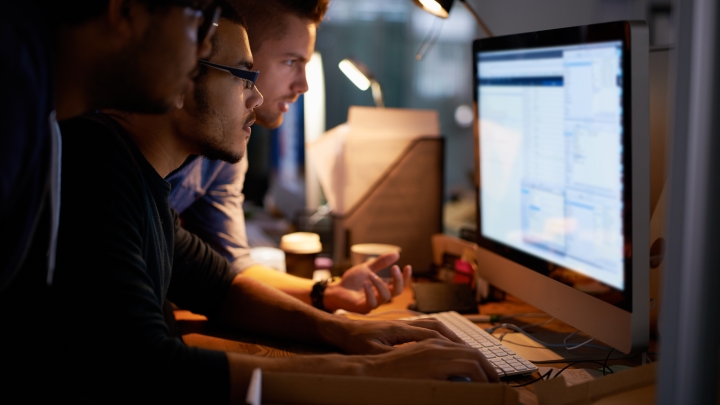Three men are intensely focused on a computer screen in what appears to be an office setting. The scene resembles one from a movie, with one face being somewhat familiar. On the left, a man wearing glasses is partially obscured. The middle figure is an Asian man with glasses, a goatee, and a mustache, dressed in a blue shirt. The man on the right is a white male with brown hair. Their attention is absorbed by the large, likely Apple-based computer monitor displaying charts or reports, though the exact contents are unclear. The cluttered desk features a white keyboard, a standing folder with white papers, and a coffee cup. In the background, a blurry desk lamp shines down, adding to the serious and concentrated ambiance of the workspace. The perspective of the photo suggests the viewer is standing to the right of the men, capturing their profile view and the busy environment they’re immersed in.